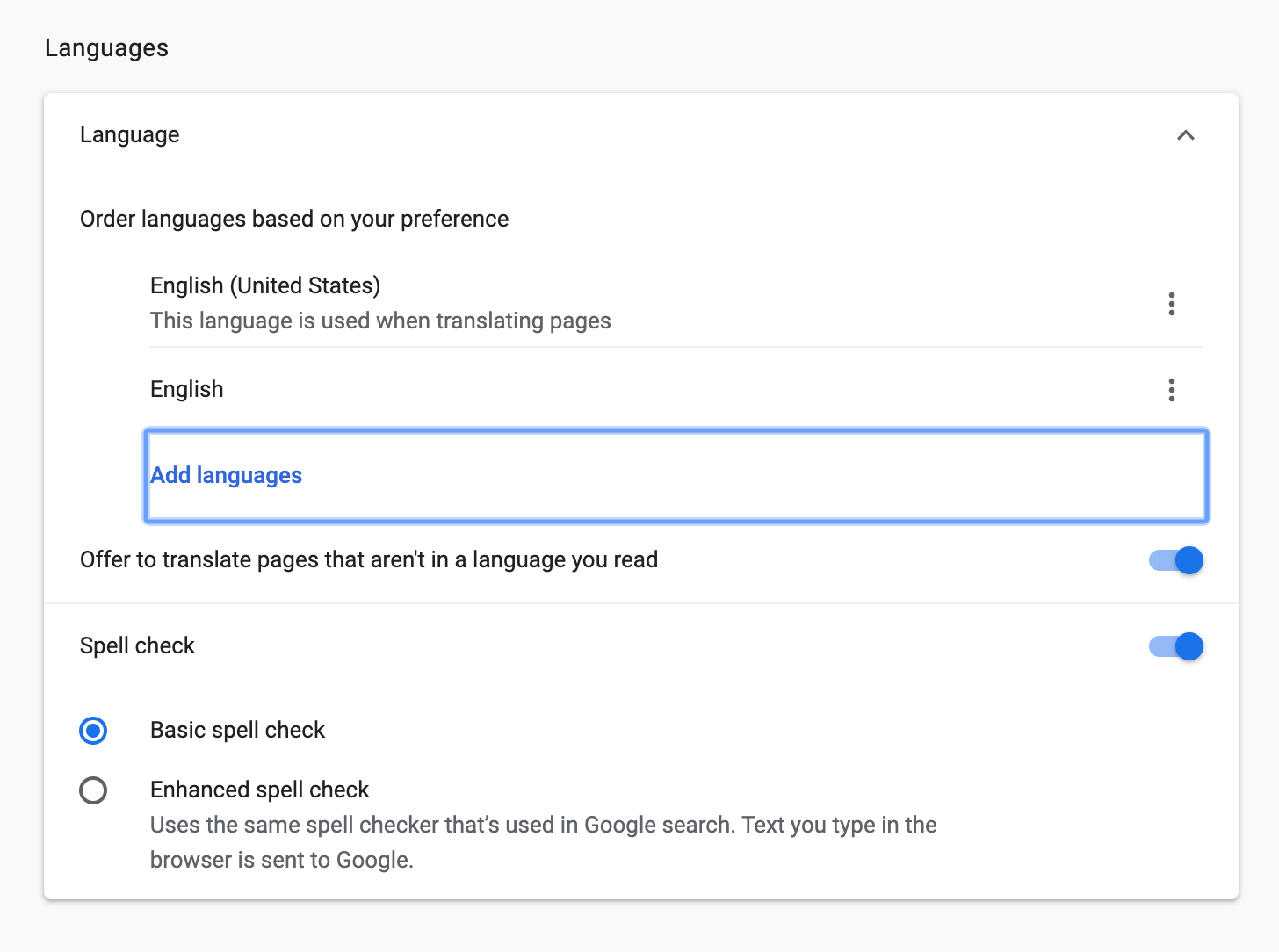The image depicts a settings section of a device, showcasing language and spell check preferences. In the background, there's a light gray square with a smaller white square layered on top. In the upper left corner of the gray square, the word "Languages" is written in black. 

At the top portion of the white square, the caption "Language" appears in black, accompanied by an arrow pointing to the top right. Beneath this, the text reads: "Order languages based on your preference," followed by "English (United States), this language is used when translating pages."

The list continues with the word "English" and the presence of an "Add languages" button, which is highlighted by a surrounding blue box. Below this, the text "Offer to translate pages that aren't in a language you read" appears in black, with a corresponding toggle indicating it is turned on.

Further down, the setting for "Spell Check" is shown, also toggled on. Within this section, "Basic Spell Check" is selected, and underneath it, a description states: "Enhanced spell check uses the same spell checker that's used in Google Search. Text you type in the browser is sent to Google."